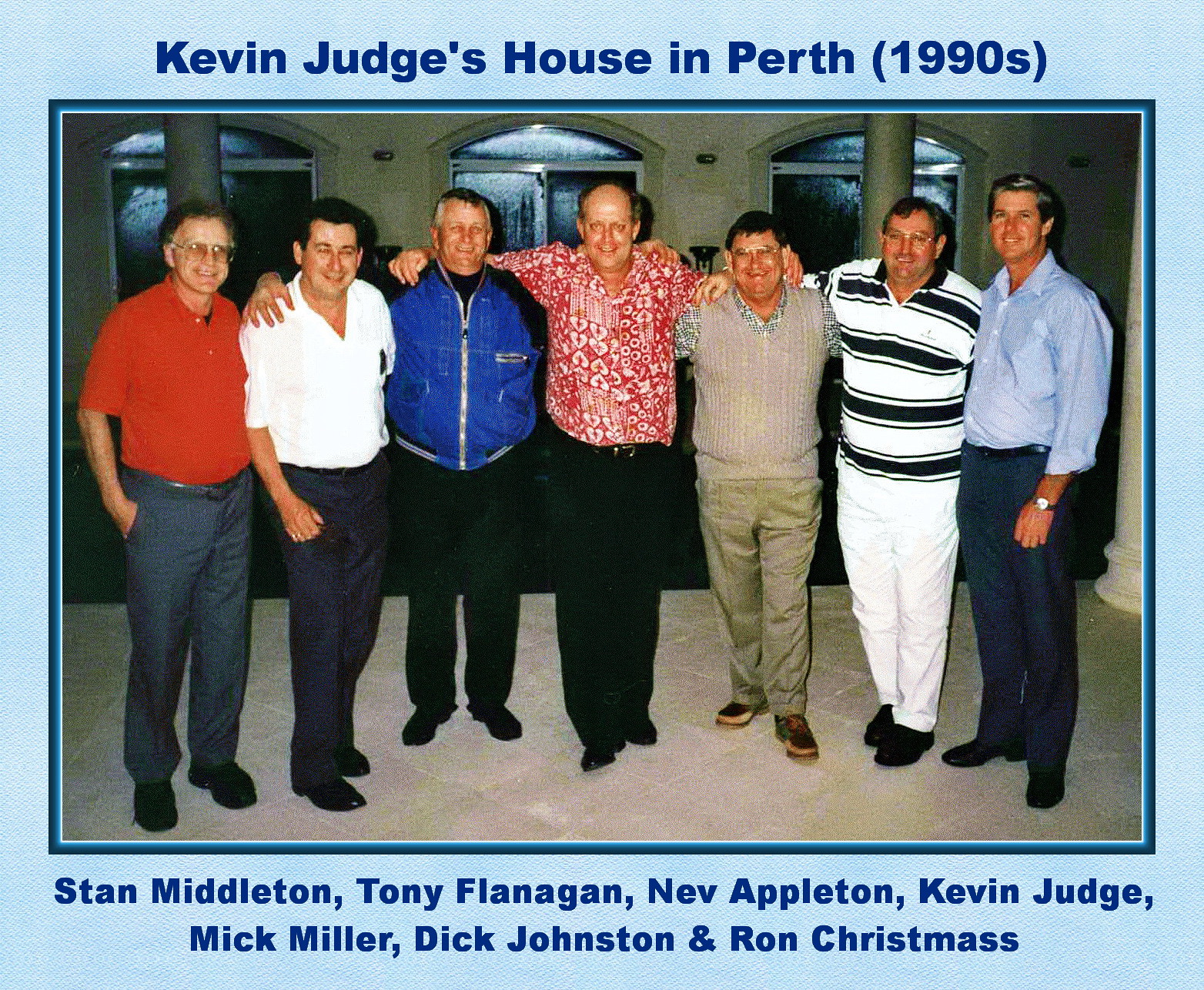The image shows a group of seven middle-aged to older men standing closely together, arm in arm around each other's shoulders, likely in a reunion setting. The image is framed by a light blue border, and at the top, in blue text, it reads "Kevin Judge's house in Perth, 1990s." Along the bottom, also in blue text, the names are listed: Stan Middleton, Tony Flanagan, Nev Appleton, Kevin Judge, Mick Miller, Dick Johnson, and Ron Christmas. The men are dressed in a mix of casual and formal outfits; for example, the man on the far right is wearing a light blue dress shirt, blue dress pants, and black dress shoes, while the man next to him dons a white shirt with horizontal black stripes, white dress pants, and black dress shoes. All the men are smiling warmly at the camera, exuding a sense of camaraderie and joyful reunion.